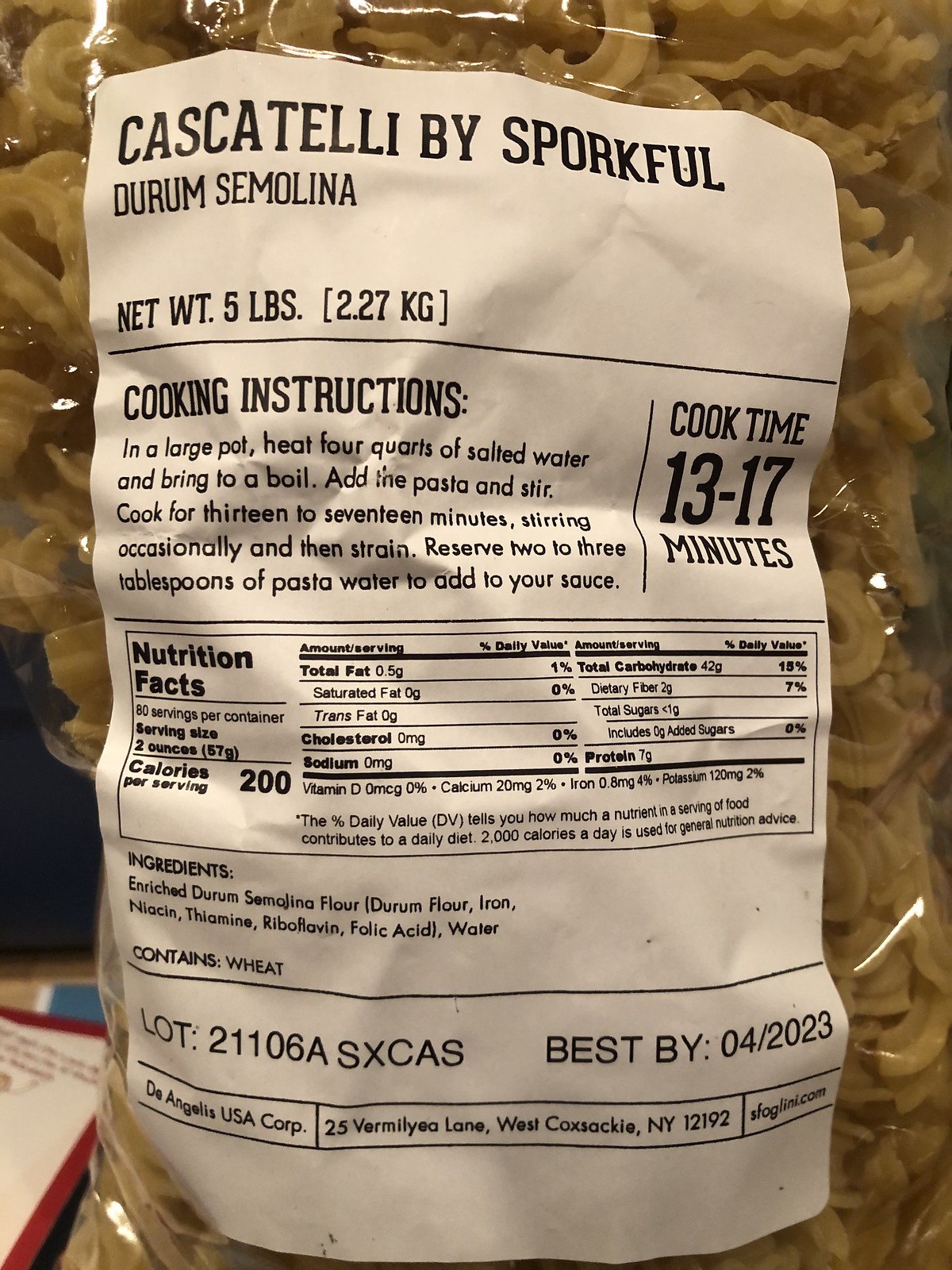This image features a close-up photograph of the back label on a clear plastic cellophane bag of Cascatelli pasta by Sporkful. The focal point is the white rectangular label prominently displayed at the center, detailing essential information against a backdrop of pasta visible around the edges. The pasta, made from durum semolina, weighs 5 pounds (2.27 kilograms). The cooking instructions advise using a large pot with 4 quarts of salted water brought to a boil, adding the pasta, and stirring occasionally for 13 to 17 minutes before straining, while reserving 2 to 3 tablespoons of pasta water for the sauce. Additional details on the label include the nutrition facts, ingredients, the corporation's address, and a best-by date of 04-2023, along with a lot number 21106ASXCAS.